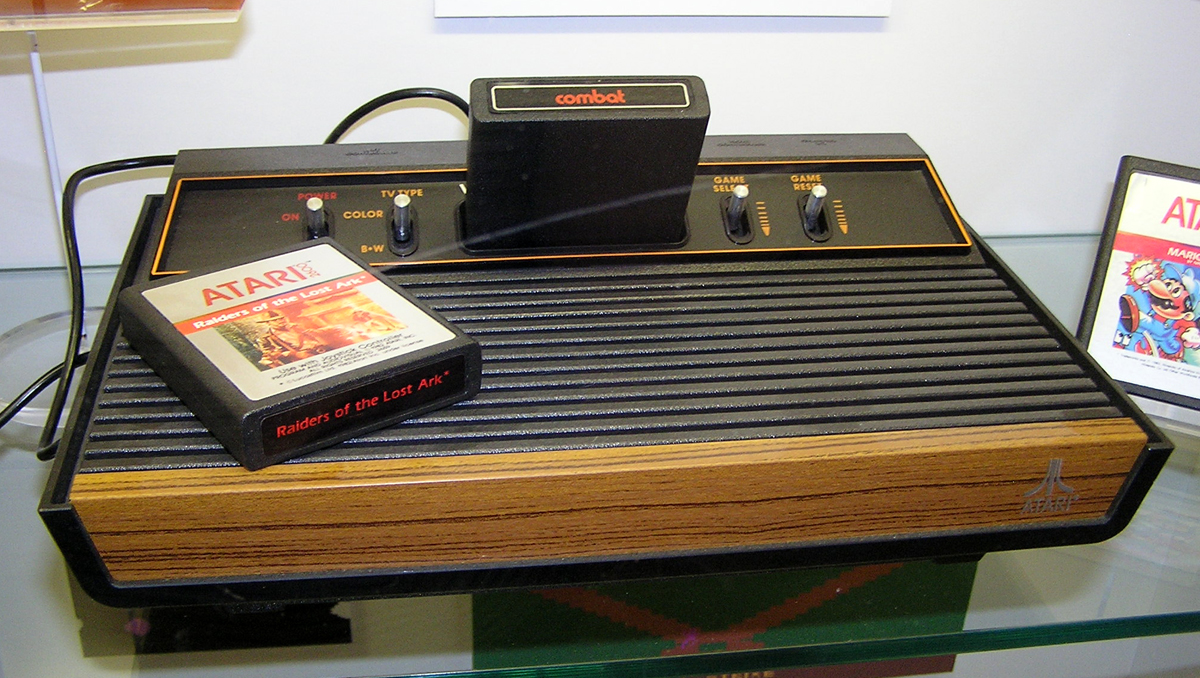The image depicts an early 1980s Atari video game system placed on a clear glass table surface. The prominent Atari console is black, with a distinct wood grain front. It features several silver knobs on top, labeled "Game Select," "Game Reset," "Power On," and "TV Type," which has options for "Color" and "BW" (black and white). The "Power On" label is in red. A protruding black cartridge labeled "Combat" in red is inserted in the middle slot of the console.

To the right of the console lies an Atari game cover, recognized by the red Atari logo. The cover showcases a Mario character—Mario is depicted wearing a blue hat and overalls, a red shirt, and white gloves, indicating it's likely a cover for a Mario-related game. Central to the image is another game cassette, "Raiders of the Lost Ark," marked by a red inscription and also branded with the Atari logo. 

Underneath the glass table, a green and brown object is visible. The backdrop is a white wall featuring some cords. Overall, the composition emphasizes the distinct vintage aesthetic of the early 1980s gaming culture.